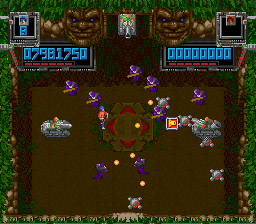Caption: 

"In this high-intensity space battle video game, the player's score is soaring past 7 million, well on its way to 8 million points. The game features a dramatic outer space setting with various ships engaged in combat. The ships, predominantly gray with glowing red lights, are interspersed with smaller purple vessels. Curiously, a humanoid figure stands prominently amidst the clash, adding an intriguing element to the scene. The score display, highlighted in blue, is organized into small boxes at the top of the screen, but some details remain unreadable. Yellowish-red projectiles are seen firing between ships, indicating active combat. Although the exact objective of the game remains unclear, the action-packed visuals suggest a strategic and thrilling battle."